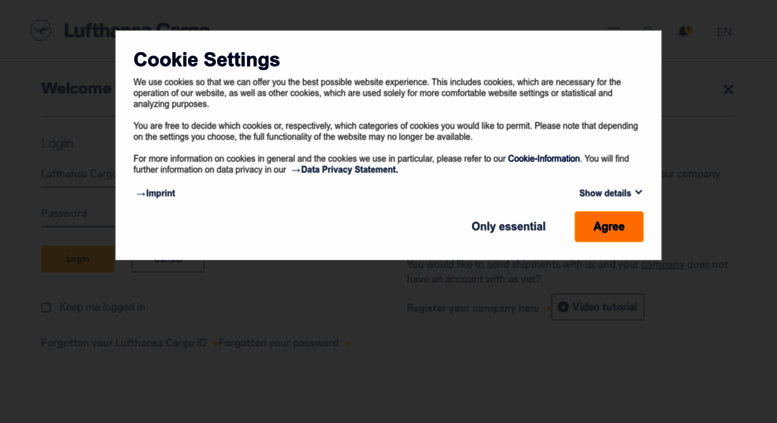The image shows a pop-up bar overlaying the original webpage. The background webpage features a dark gray color and is partially visible behind the pop-up. Some discernible elements from the background page include the words "welcome," "login," "one time password," and a yellow "login" button. Additionally, phrases such as "keep me logged in," "forgotten your login," "forgotten your password," as well as "video tutorial" and "register your company here" are present, suggesting it is a login or registration page for shipment management.

The central focus is the white pop-up box with the header "Cookie Settings." This box explains the company’s cookie usage policy. The phrase "Cookie Settings" is prominently displayed in large blue letters. Within the explanatory text, terms like "cookie information," "data privacy statement," "imprint," "show details," and "only essential" are highlighted in a darker blue coloration. In the bottom right corner of the pop-up, there is a yellow rectangular button with the word "Agree" written in black, inviting the user to accept the cookie policy.